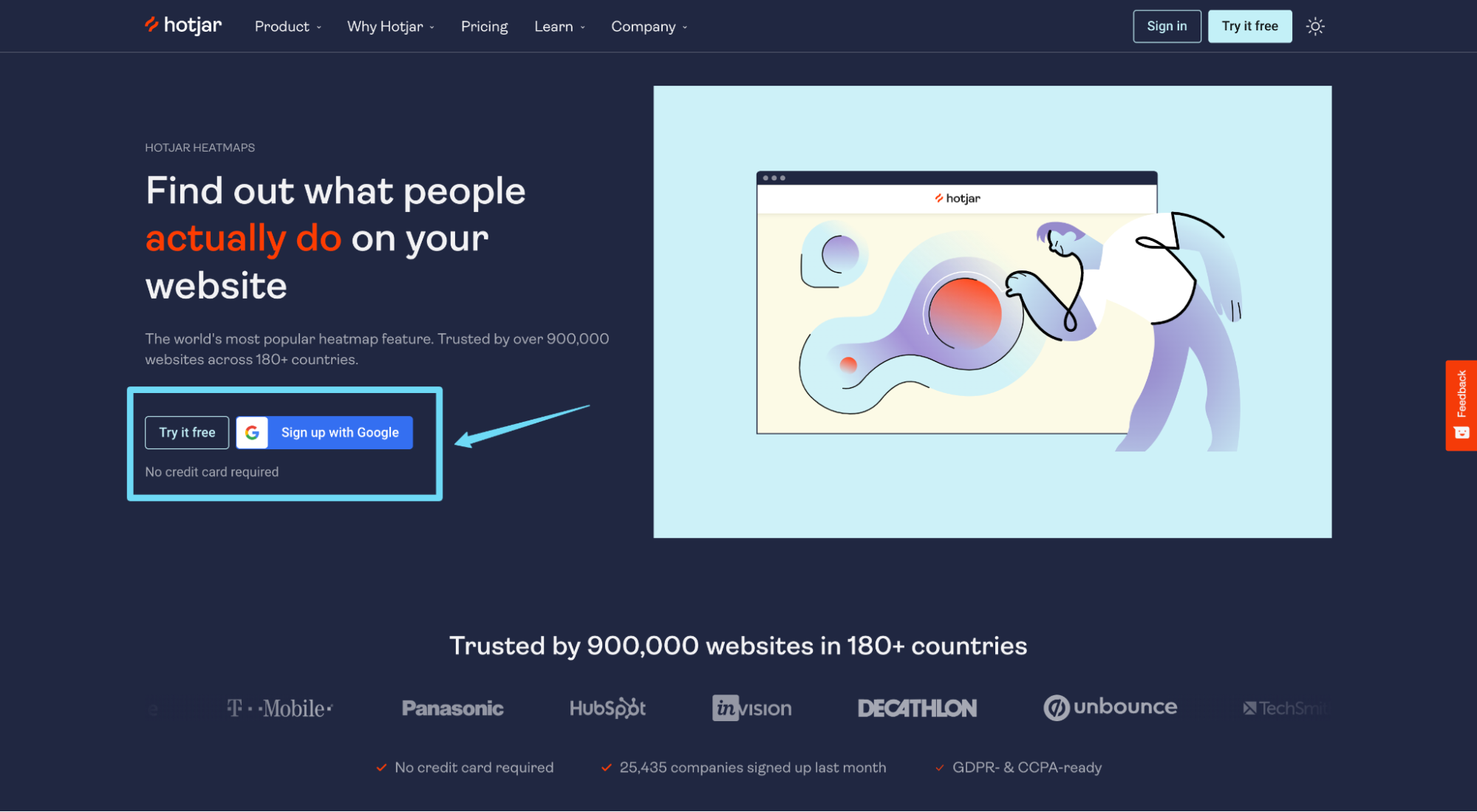The image depicts a webpage on the official website for Hoja, a popular heatmap feature used for website analytics. The top navigation bar includes labels such as "Products," "Why Hoja," "Pricing," "Learn," and "Company." Prominently, the slogan "Find out what people actually do on your website" is displayed alongside a brief description, "World's most popular heatmap feature, trusted by over 900,000 websites across 180+ countries."

There are options to "Try it free" and a button to "Sign up with Google," which emphasizes that no credit card is required for sign-up. On the right side of the page, the Hoja logo is visible. Below these elements, additional text reiterates Hoja's trustworthiness: "Trusted by 900,000 websites in 180+ countries," followed by logos of notable companies such as T-Mobile, Panasonic, HubSpot, Envision, Decathlon, and Unbounce.